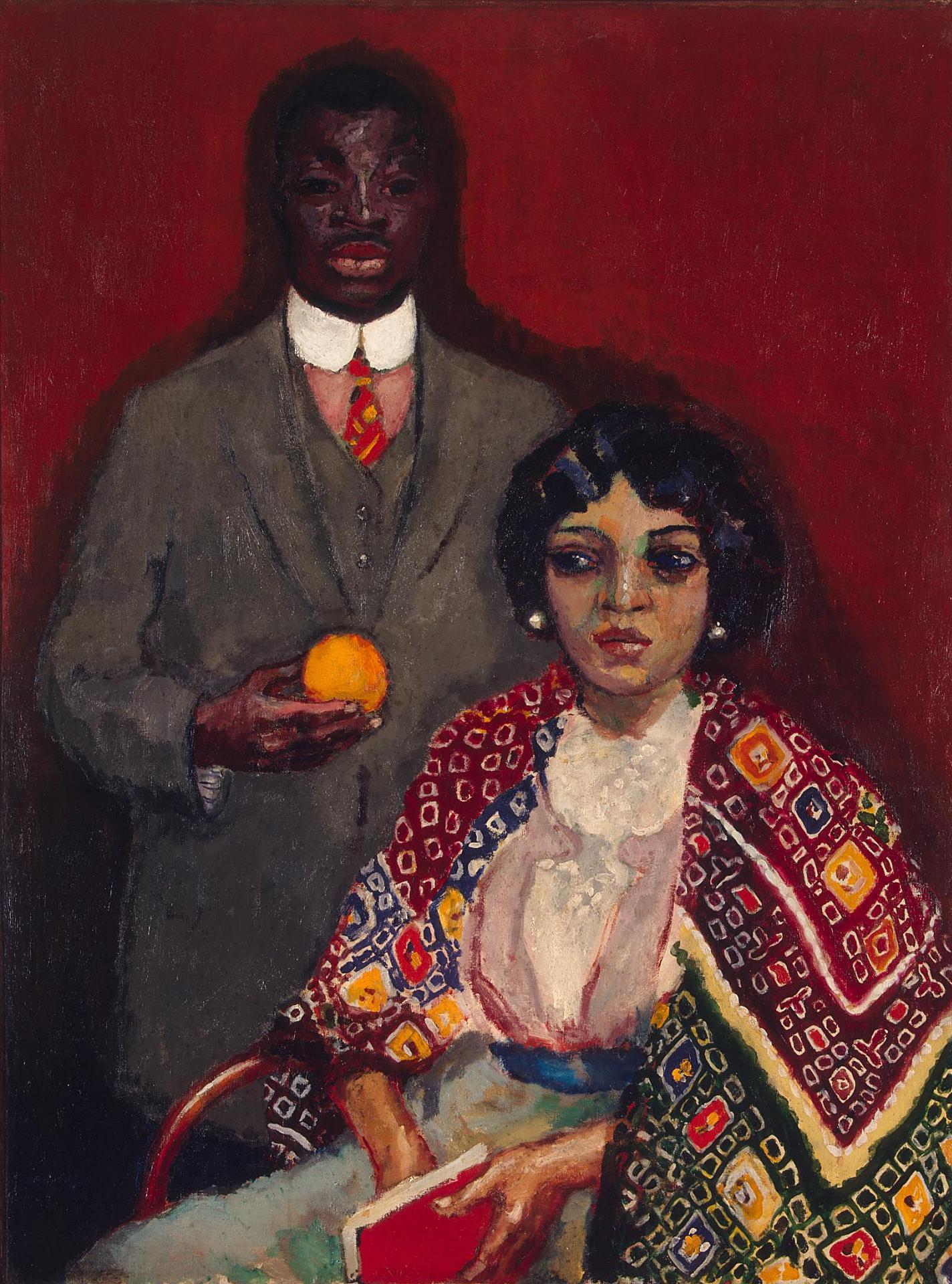The painting depicts an elegant African-American couple, with the light-skinned woman seated on a wooden chair, holding a book in her hands. She's adorned in a vibrant, multi-patterned shawl featuring colors like red, green, and blue, which complements her white dress and blue sash. Her dark hair is accessorized with two earrings, and she gazes contemplatively to the right side of the image. Beside her, partially in the background, stands a darker-skinned man, dressed in a brown suit with a striking red and yellow tie. He holds an orange in his right hand against a vivid orange-red background. Both figures have neutral expressions, adding to the painting's enigmatic allure. The painting, rich with colors—red, orange, yellow, green, blue, burgundy, gray, black, white, light blue, brown, beige—captures an upper-class aura and is set within a vertical rectangular frame.